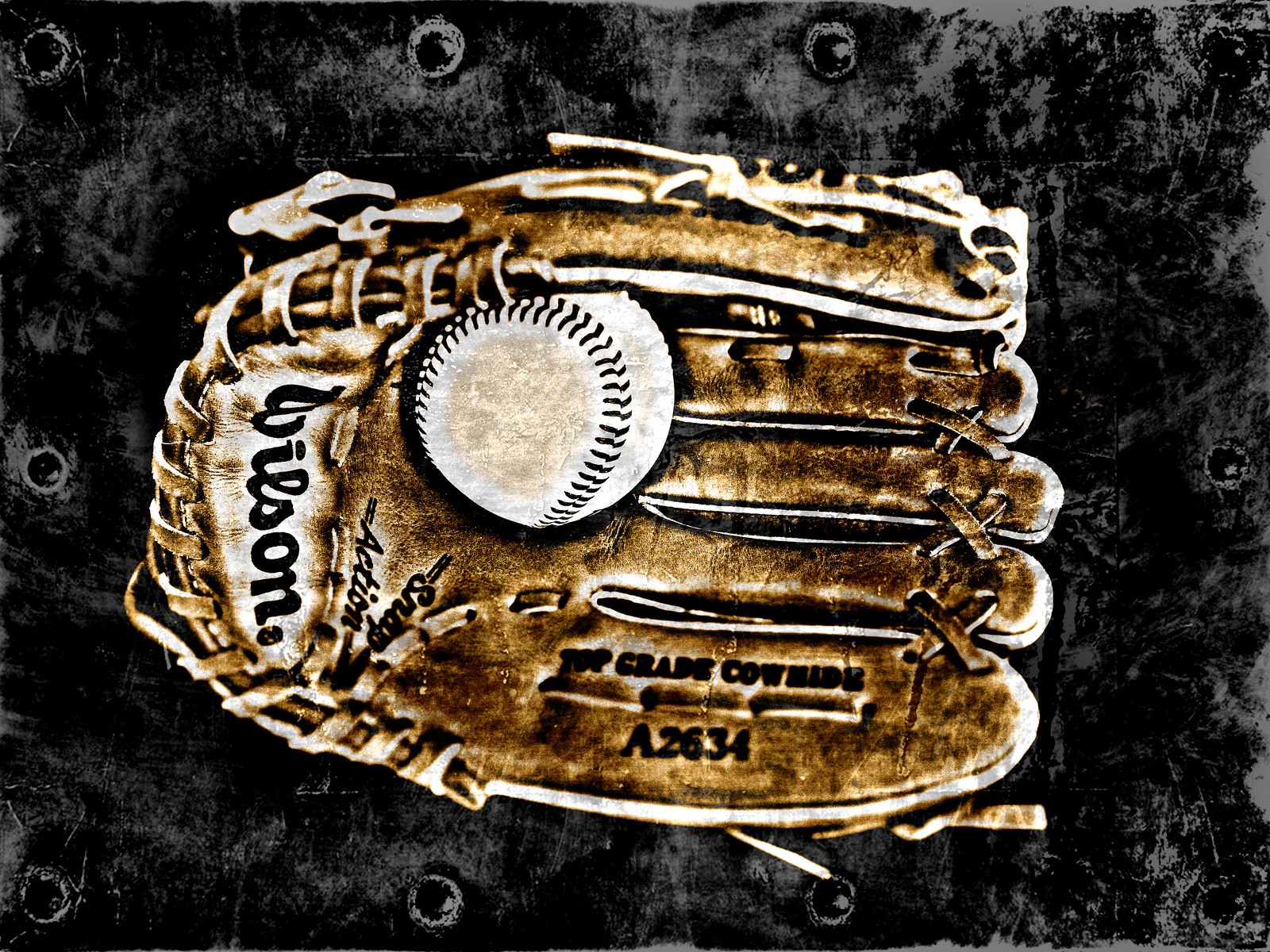The image depicts an edited photograph of a Wilson baseball mitt holding a baseball at its center. The mitt, crafted from top-grade cowhide and marked with the serial number A2634, appears in a faded brown tone, suggesting either artistic effects or age. The photograph exudes a high level of contrast and utilizes multiple filters, giving it a bright, dried-out appearance. The background of the image is a rich, black velvet material, providing a stark and elegant contrast to the subject. The baseball mitt is positioned horizontally with the glove open to the right, prominently displaying its hand-sewn leather stitching. A white baseball rests securely in the middle of the mitt, completing the composition. No people, dates, or additional text are present in the photograph, maintaining a focused and timeless quality.